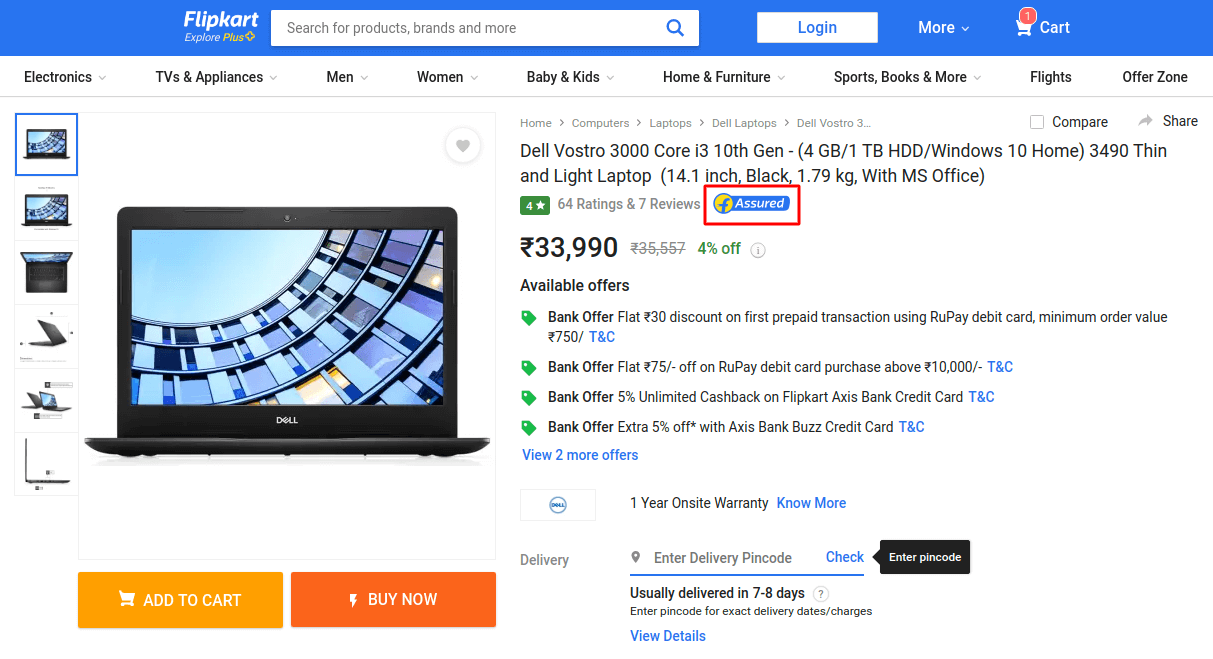The screenshot features the Flipkart website with a prominently displayed "ExplorePlus" section. The background of the site is white, while the top navigation bar is blue. This top bar includes options such as searching for products, brands, and more. It also features buttons for login, additional options, and a cart icon indicating one item in the cart.

Below the navigation bar, categorical options are listed: Electronics, TV and Appliances, Men, Women, Baby and Kids, Home and Furniture, Sports, Books, More (with a dropdown), Flights, and Offer Zone.

The main content area showcases a laptop advertisement for the Dell Vostro 3000. Detailed specifications of the laptop include:
- Intel Core i3 10th Gen processor
- 4GB RAM
- 1TB hard drive
- Windows 10 Home Edition
- Model: 3490 thin and light
- 14.1-inch display
- Color: Black
- Weight: 1.79 kilograms
- Includes Microsoft Office

The laptop is priced at 33,990 yen, reflecting a 4% discount. The page also highlights various bank offers that provide additional savings on the purchase. Below the product details, there are buttons for "Add to Cart" and "Buy Now" for convenient purchasing options.